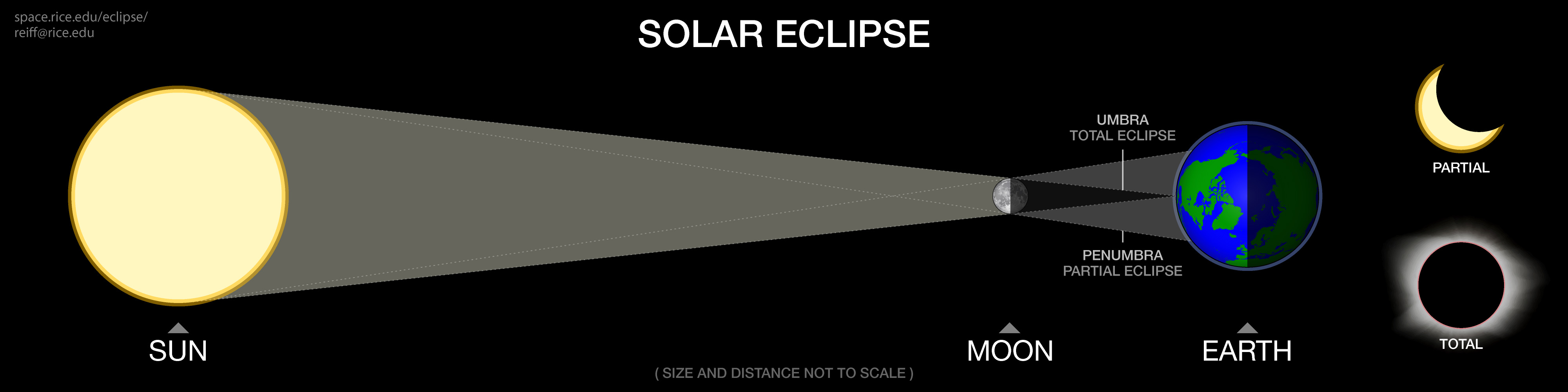The image is a detailed diagram of a solar eclipse on a long, rectangular black background. At the top center, "SOLAR ECLIPSE" is written in bold, white capital letters. On the left side of the diagram, there is a yellow circle labeled "Sun." The sunlight projects across the diagram, illuminating the moon, which is situated in the middle. The moon shows a clear contrast between the lit side, illuminated by the sun, and the dark side. Two triangular sections extend from the moon towards the Earth, demonstrating the different kinds of eclipses. The upper triangle, labeled "Umbra, Total Eclipse," indicates the area experiencing a total eclipse, while the lower triangle, labeled "Penumbra, Partial Eclipse," signifies the partial eclipse region. The Earth, depicted in blue with green continents, has half of its face lit up and the other half in darkness.

On the right side of the image, there are two smaller illustrations. The top illustration shows a partial eclipse, making the sun appear as a yellow crescent. Below it, the illustration of a total eclipse features a black circle surrounded by a white halo of light. The bottom part of the diagram includes a note in gray text, stating "Size and distance not to scale." This comprehensive, high-contrast visual guide effectively conveys the mechanics and visual appearance of a solar eclipse.